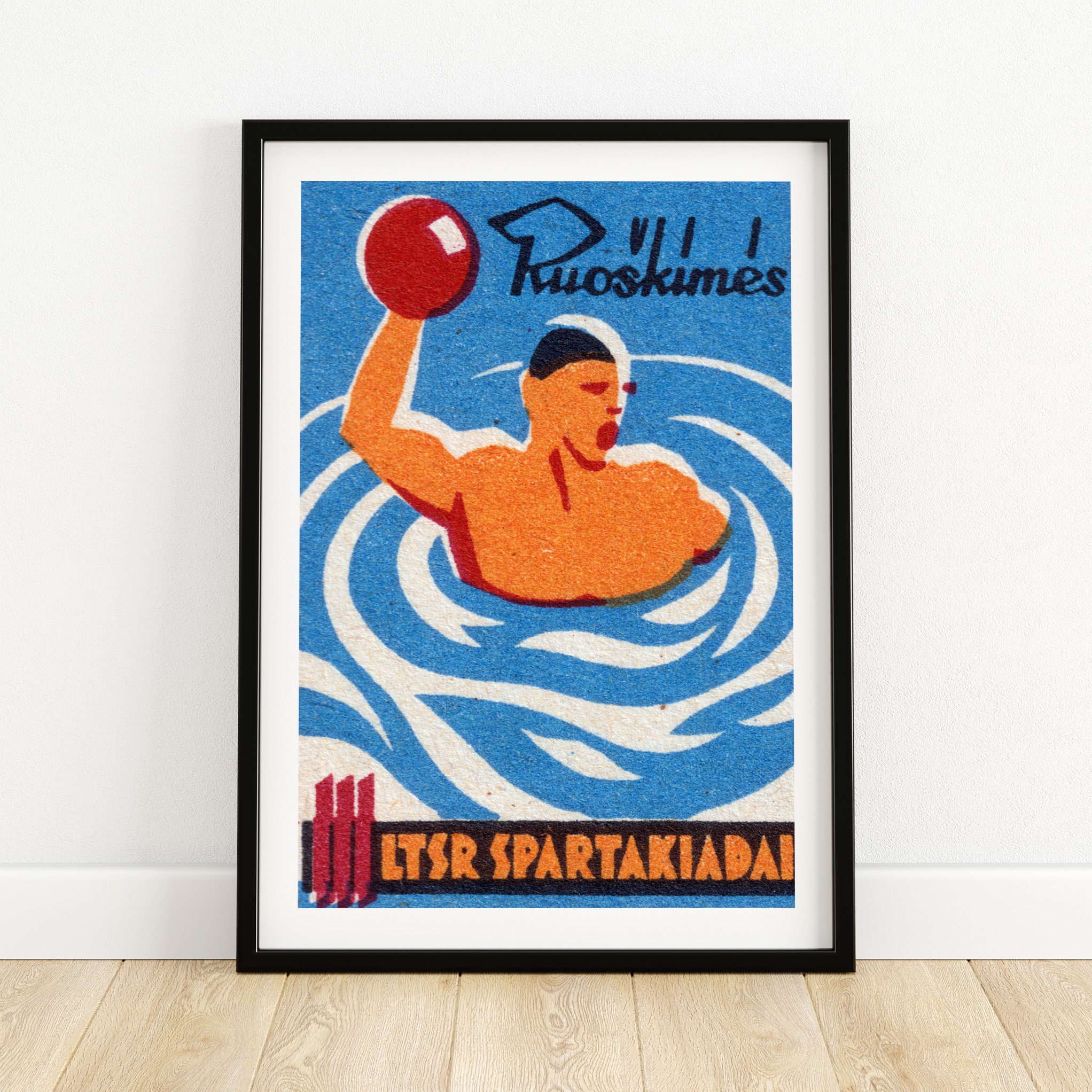The image portrays a color photograph of a framed poster leaning against a white wall on a light gray or brownish beige wooden floor. The poster, encased in a black frame with a large white border, showcases a stylized, simple drawing of a man playing water polo. The man, wearing a black swimming cap and facing to the right, holds a red ball in his right hand. The background of the image features swirling blue and white hues to represent moving water with ripples around the figure. At the top of the poster, the word "RUOSKIMES" is displayed, followed by a symbol resembling a "V" and two vertical lines. At the bottom, three red vertical lines precede the text "LTSR SPARTAKIADA," though the last letter is not fully visible. The writing appears to be in a foreign language, potentially Russian. The tagline at the top is in dark blue, while the bottom tagline is in bright orange, creating a contrast against the mostly blue-toned image.